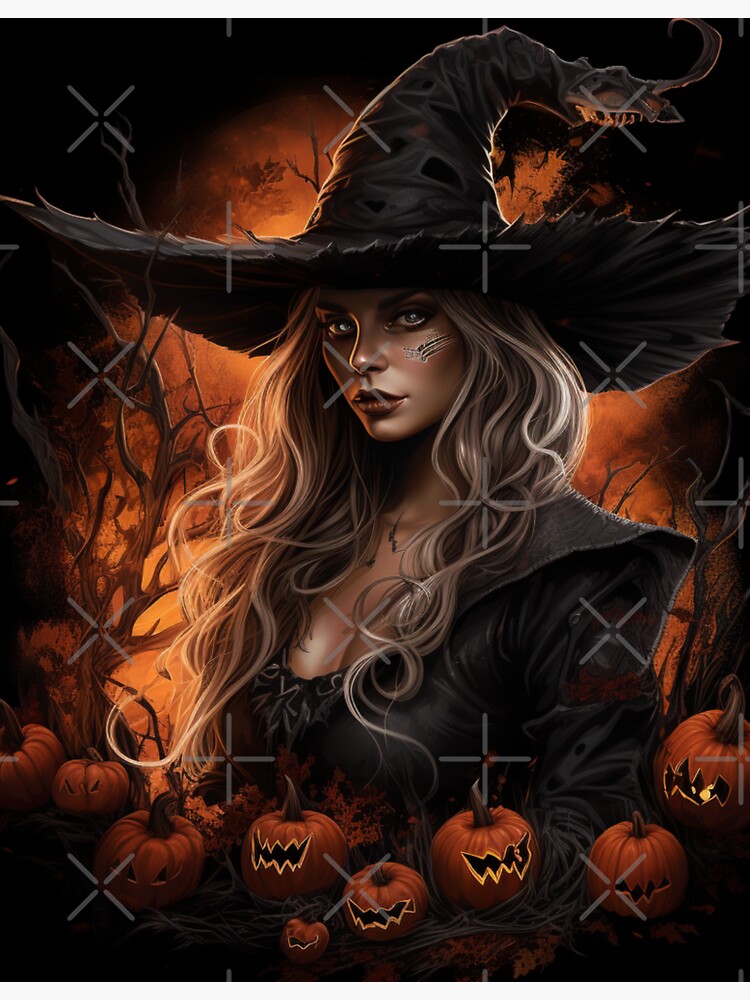This digital artwork vividly depicts a young, enchanting witch exuding a Halloween theme. Her striking appearance is defined by a large, wide-brimmed black witch's hat that curves back stylishly. She has long, flowing blonde hair that cascades down, almost like extensions, adding to her captivating charm. The witch's face is illuminated, almost glowing, accentuated by her radiant white skin and the orange outline behind her. Her makeup is meticulously detailed, with expressive lipstick and a unique pattern resembling three scratches beneath her eye. She wears a sexy witch’s outfit, a black, low-cut jacket with pointed shoulders that reveals her cleavage and cuts off near her breasts. In the foreground, a collection of eerie jack-o'-lanterns are visible, some carved with toothy grins and others adorned with black designs. The background features ominous dead trees and an evocative fiery orange glow, reinforcing the spooky, Halloween atmosphere of the piece.